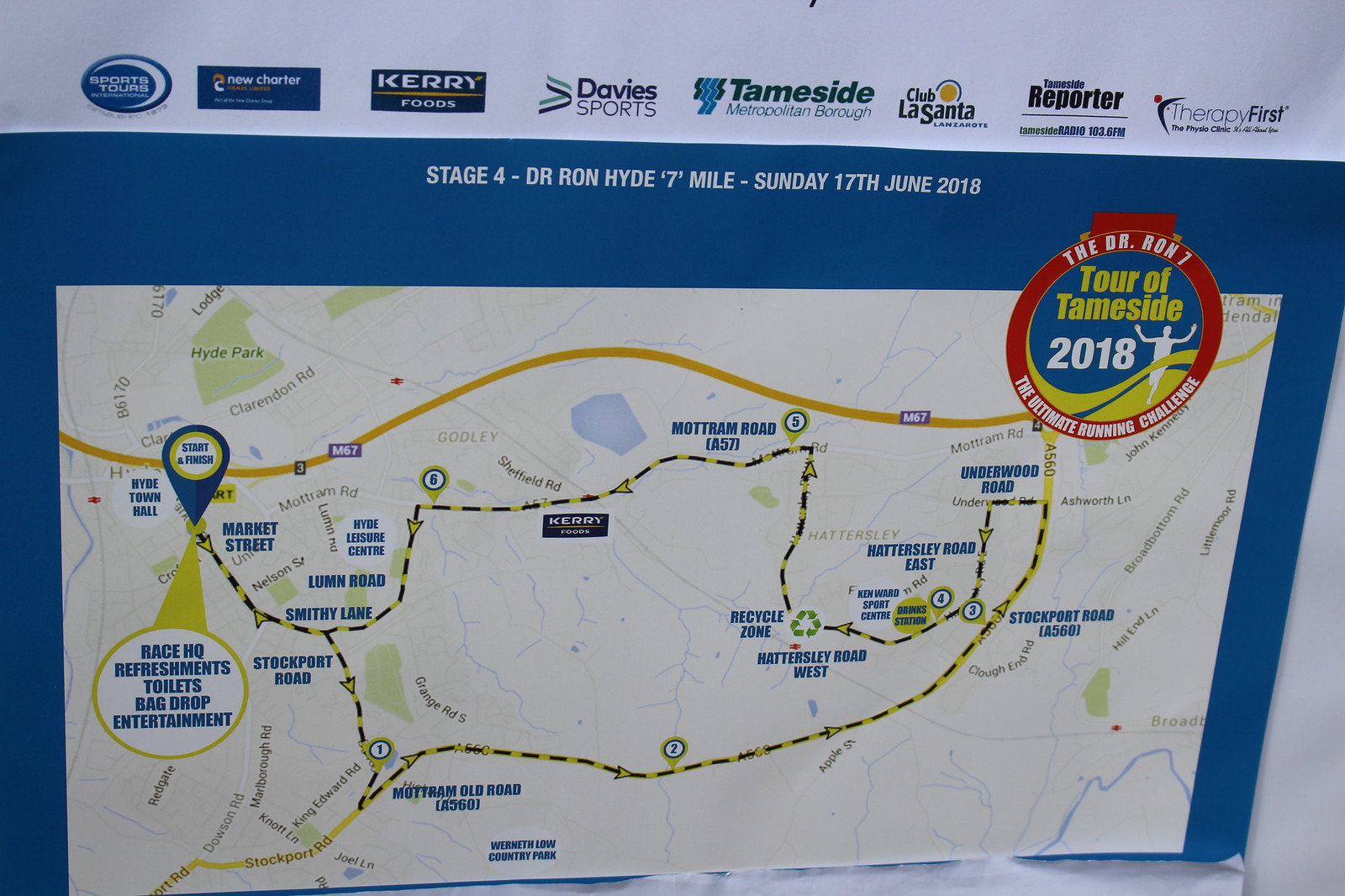This wide rectangular image showcases a map on a sign, which is cut off at the bottom left corner, affixed to a white wall. At the top of the sign, an off-white banner features several logos from companies including Sports Tours, New Charter, Kerry Foods, Davie Sports, Tameside Metropolitan Borough, Club La Santa, Tameside Reporter, and Therapy First. The map, bordered by a dark blue section at the top, prominently displays the text "Stage 4, Dr. Ron Hyde, 7 Mile, Sunday 17th, June 2018" in white lettering. Additionally, a circular logo on the right reads "Tour of Tameside 2018" and includes an image of a person running on a track. The map details a large area, indicating the path for a 7-mile run, along with landmarks such as Race HQ, refreshments, toilets, bag drop, entertainment, and the start/finish line, marking it as part of a running challenge event.